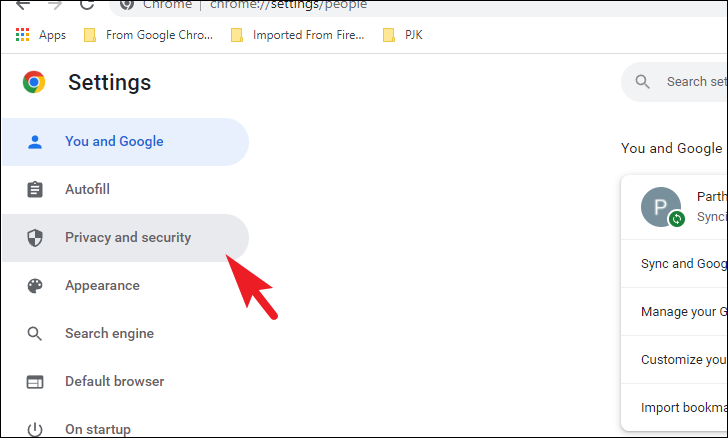A cropped screenshot of a web browser displaying the Chrome settings page. The image captures the top portion of the browser, where the search bar is partly visible, with half of it edited out. The title "Chrome Settings" is shown prominently next to the "People" section. Beneath this, the main tab is open to the "Settings" menu.

On the left side, a vertical list of settings options is displayed. At the top of this list, the word "Settings" appears in large black letters, accompanied by the Chrome icon to its left. The first option, "You and Google," is highlighted in blue, while the third option, "Privacy and Security," is highlighted in gray. A red arrow has been edited into the screenshot, pointing directly at the "Privacy and Security" option. 

Below "Privacy and Security," additional categories include "Appearance," "Search Engine," "Default Browser," and "On Startup," although the list is truncated. On the right side of the image, the top-right search bar is partially cropped out, and just below it, "You and Google" text is visible along with part of a white panel, with the rest being cropped out of the frame.